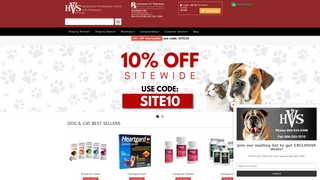**Detailed Caption for Website Image:**

The image showcases a website dedicated to pet care. The logo, "HVS," is prominently displayed at the top left corner of the page, featuring a larger "V" within a reddish banner. To the right of the logo, there's an orange button and a search bar located directly underneath the "HVS" emblem. Beneath these elements is a black navigation bar with various links.

The main content area of the page is white and features a promotional banner announcing "10% off site-wide," with the discount code "SITE10" highlighted in a red box. Adjacent to this text are images of a dog and a cat. The dog has floppy ears, a predominantly brown face with a white midsection, and black eyes. The cat, primarily white, has distinct gray markings on its face.

On the bottom right of the page, there's another image showing a bulldog accompanied by text featuring "HVS." Additionally, the lower section of the page displays various pet products categorized under "Dog and Cat Best Sellers." The products include items such as Heartgard, depicted as red and green pills, alongside smaller bags positioned to the left.